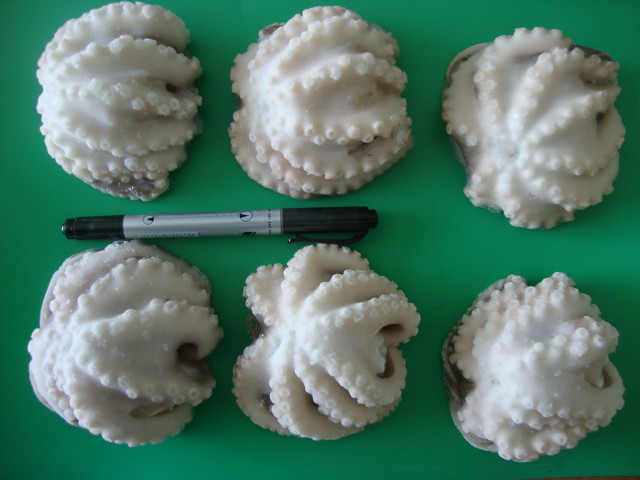This photograph captures a top-down perspective of six white, spherical sculptures with tentacle-like extensions, closely resembling baby octopuses or small squids. Positioned on a flat, pale green table, the sculptures are arranged in two neat rows of three. These round structures are detailed with small, circular dots mimicking suction cups, enhancing their lifelike appearance. The color of the sculptures is predominantly pearl white with subtle shades of dark purple and hints of gray, possibly influenced by the lighting or flash used in the photo. A black marker with a silver middle segment is placed horizontally between the first four sculptures, adding a stark contrast to the otherwise minimalist setting. The scene is enclosed within a square frame, emphasizing the orderly placement and uniformity of the objects.